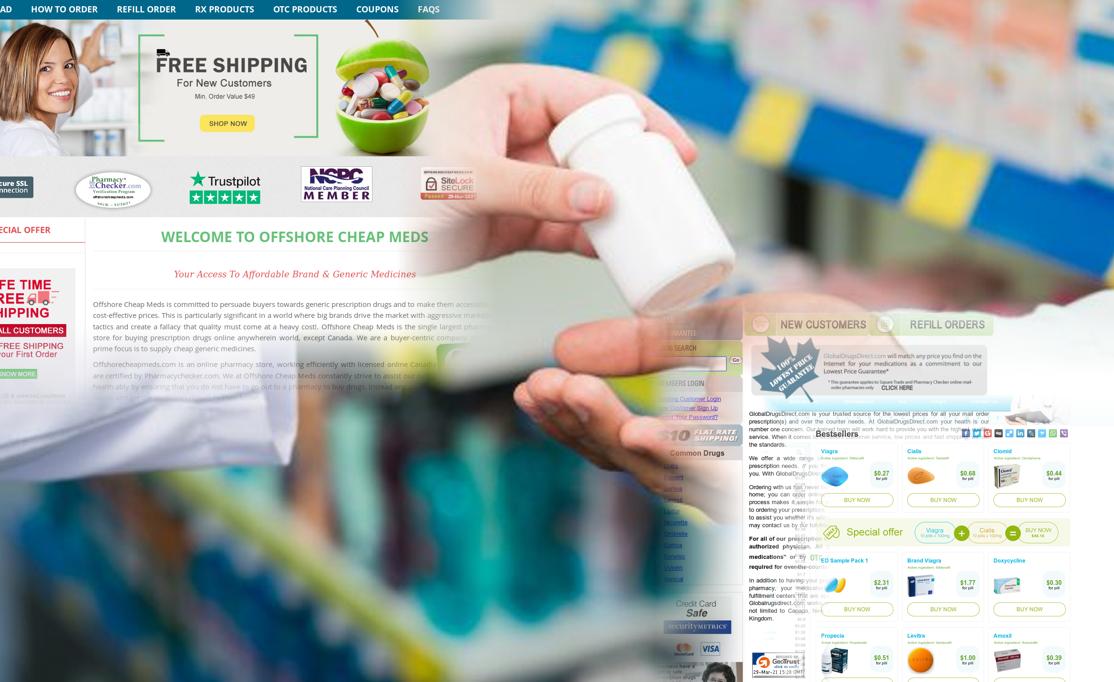The website "Welcome to Offshore Cheap Meds" prominently features a pharmacist smiling at the camera while holding a pill bottle. At the top of the site, a blue header displays navigation options such as "How to Order," "Refill Order," "RX Products," "Over-the-Counter Products," "Coupons," and "FAQs." Centered on the page in bold, green capital letters is the site's welcome message. Additionally, a promotional banner with a green border and a small black truck icon offers free shipping for new customers on orders over $49.

To her side, an image of an apple filled with prescription medicines is displayed, emphasizing the health focus of the website. The homepage proudly showcases a five-star Trustpilot review, reinforcing its credibility. Below the welcome message, the site highlights its commitment to providing access to affordable brand-name and generic medications, underscored by red letters announcing free shipping on the first order.

Further down, the page features a variety of offers on best-selling medicines, complete with images and prices. The background image of a pharmacist handing a bottle of medication to a customer ties everything together, illustrating the site's dedication to customer service and the accessibility of affordable healthcare solutions.